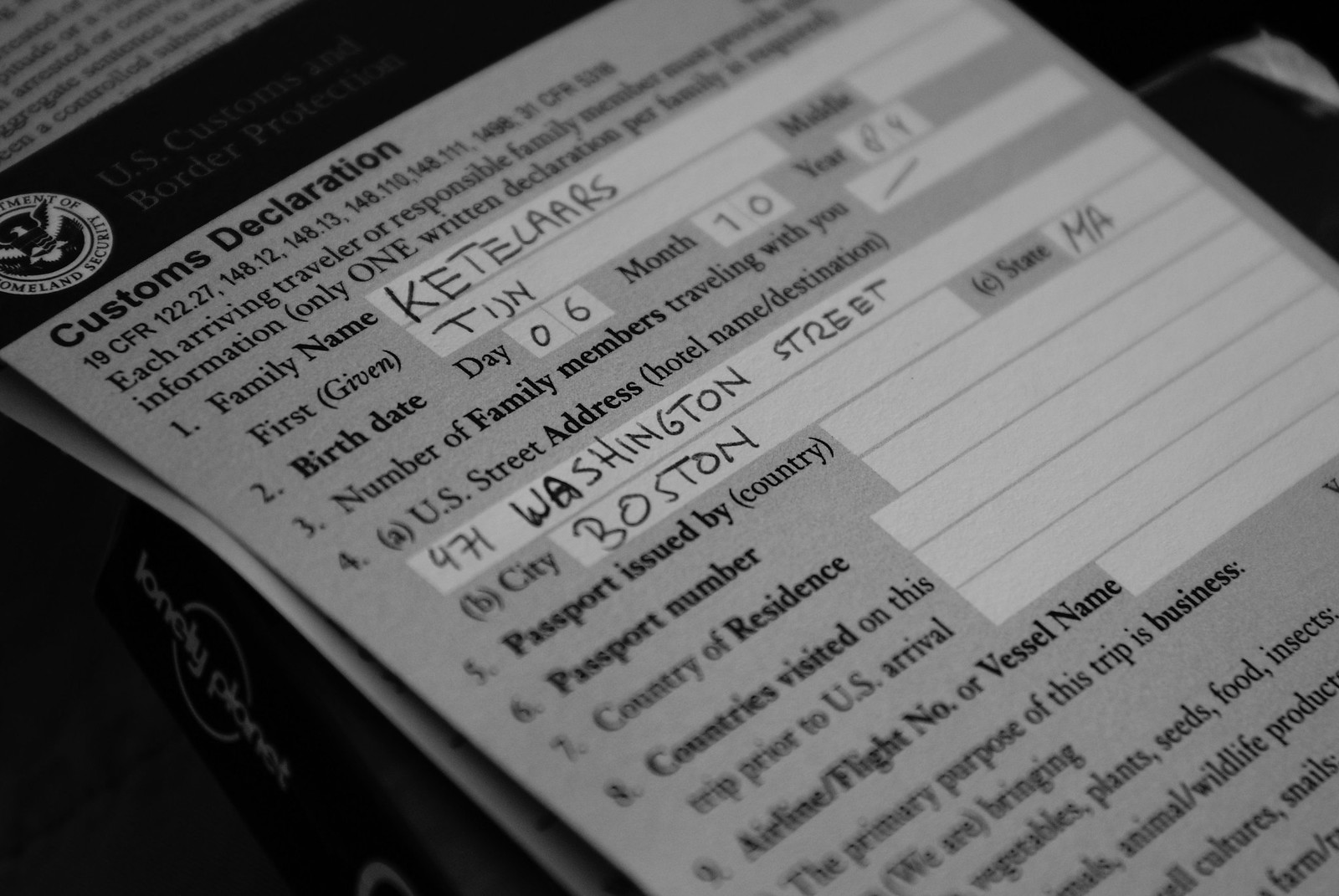The image depicts a black-and-white photograph of a U.S. Customs and Border Protection form titled "Customs Declaration." The form, viewed at an angled perspective with the top left corner pointing upward, features prominently in bold black font the text "Customs Declaration" followed by "19 CFR 122.27, 148.12, 148.13, 148.110, 148.111". Below this, several lines are blurred but can be partially deciphered to read, "each arriving traveler or responsible family member" and "Information (only one written declaration per family)." There is a visible Homeland Security emblem in the top left corner, suggesting the form pertains to documenting travel information. The form includes fields for family name, birth date, number of family members, city, address, passport, and vessel, indicating its use for international arrivals, possibly those arriving by boat. The lower section of the form contains multiple white boxes intended for handwritten information.